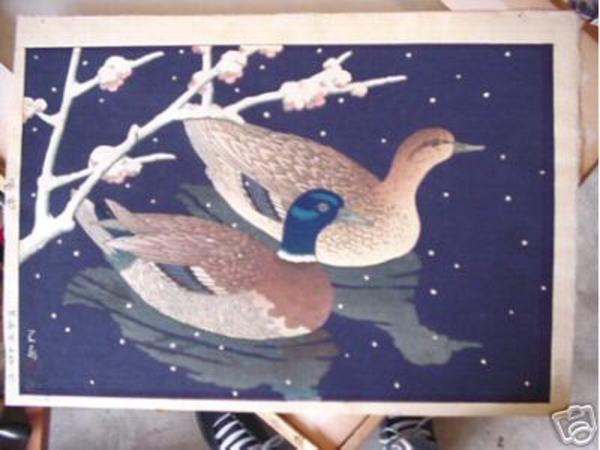A framed photo, likely taken with a phone due to its casual composition and poor quality, captures two ducks or possibly mallards swimming in a dark navy blue lake dotted with white circles. These circular spots, resembling fallen petals, are reflected along with the ducks and a tree branch extending over the water. On closer examination, the ducks' details suggest one is a male mallard, distinguished by its traditional green head, white neck ring, and colorful plumage, while the other appears to be a browner, less extravagant female. The scene is set at night, with star-like reflections visible on the water. The wooden frame is of a light-colored wood, and in the bottom corner of the image, a pair of gray shoes with white laces, possibly belonging to the picture-taker, adds an unintentional but casual element to the composition.